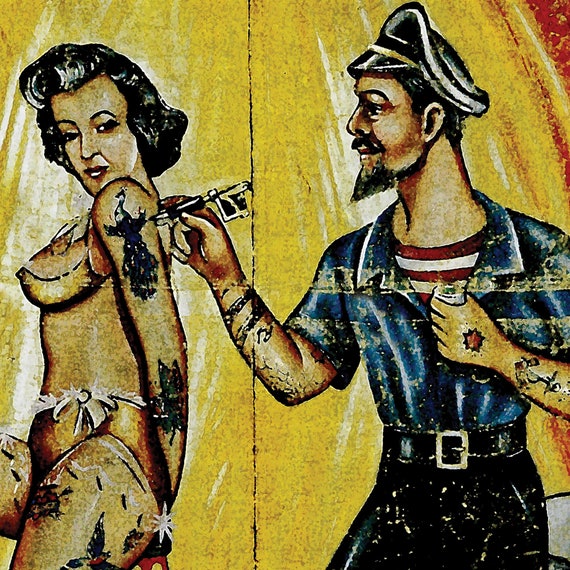This artwork is a vintage-style mural with a square format, featuring a dynamic and colorful depiction of a scene from a bygone era. The mural's background is predominantly yellow with a striking patch of red in the upper right corner, creating a vibrant setting for the characters.

Central to the image is a sailor dressed in black pants, a black belt, and a blue short-sleeved collared shirt worn over a red and white horizontally-striped shirt. He sports a goatee and wears a classic black sailor’s hat. His arms are adorned with tattoos, including an anchor and a red star on one hand. In one hand, he holds a can of beer, while his other hand meticulously tattoos a peacock design on a young woman. 

The woman, facing left with her head turned towards the viewer, exudes a vintage charm reminiscent of the 1950s, highlighted by her short, slightly curly hair that falls to the base of her neck. She is clad in a revealing yellow bikini, accentuating her voluptuous figure. Her body showcases multiple tattoos, including pieces on her thigh and forearm. The sailor’s concentration and the woman’s composed expression capture a moment of intimate artistry within this striking mural.